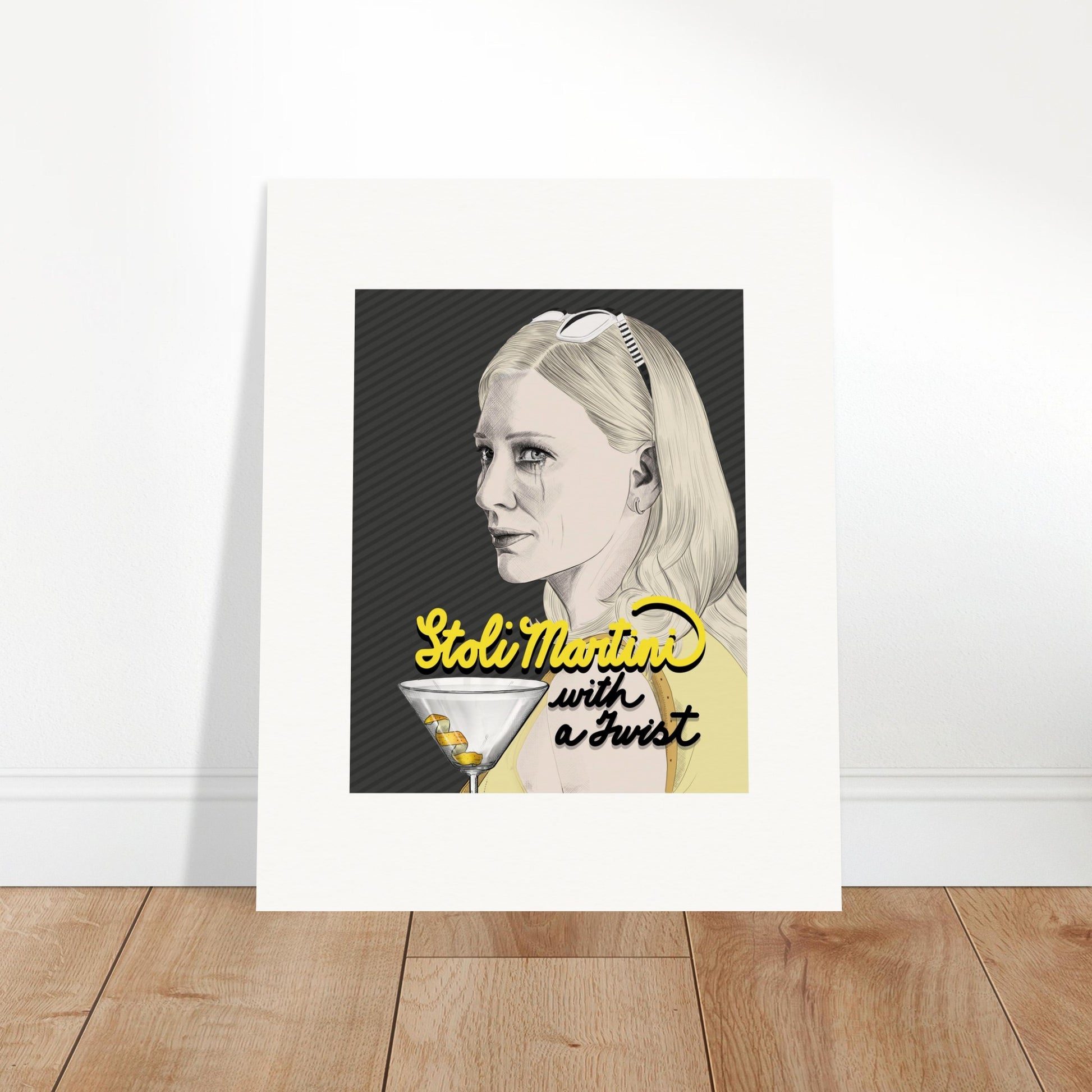The image captures a detailed scene with a white-framed photograph propped against a pristine white wall, resting on a brown hardwood floor that occupies the bottom portion of the view. The photograph within the frame features a woman with tears streaking down her face, particularly noticeable under black mascara trailing from her right eye. Her blond hair is mostly pulled back, with sunglasses perched atop her head. The background of the image behind the woman is black, accentuating her lighter skin tone. Just below her side profile, the text "S-T-O-L-I, Martini with a twist" appears in bright yellow, situated above a minimalist martini glass that contains three yellow elements. The overall atmosphere is bright and clear, likely due to ample natural lighting, suggesting the picture was taken in a well-lit, possibly museum-like environment.